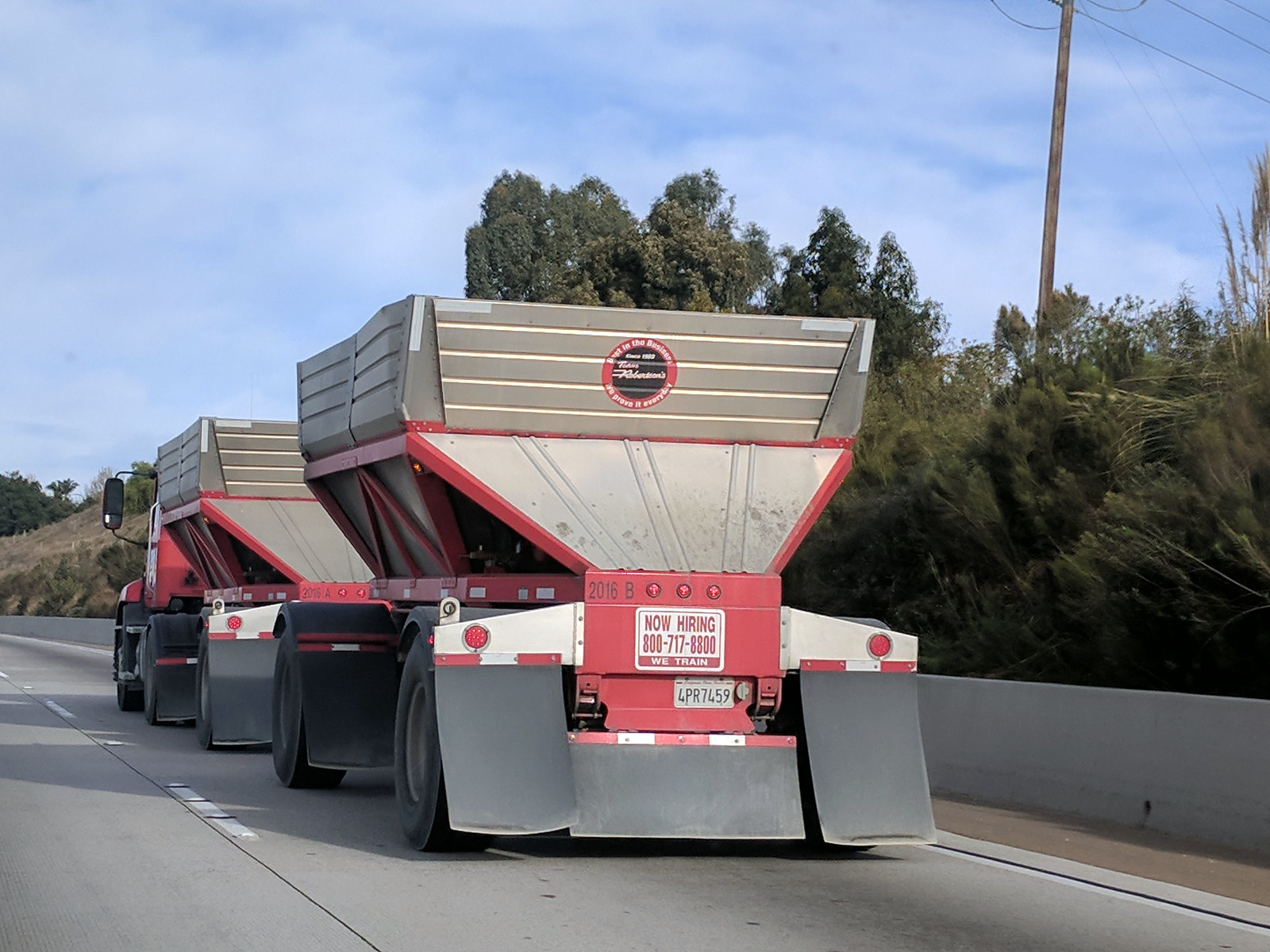The image features a large industrial truck, predominantly red and silver, with an extended truck bed. It carries two sizable steel containers with red painted borders, positioned at the front and rear of the bed. Both the containers and the bed are substantial, suggesting the truck could be used for heavy-duty purposes like a cement mixer or dump truck. The truck sits on a gray pavement road alongside a white wall, with tall green trees and bushes swaying behind it under a sunny, light blue sky dotted with some clouds. On the truck's rear, which is painted red, there is a sign that reads "Now Hiring" followed by the phone number, and below it, "We Train," all in red text on a white background. A license plate can be seen below the sign, and there is some additional unreadable writing or a logo at the top of the silver containers. The truck’s tires are large and black, with equally substantial black mud flaps extending behind each one.